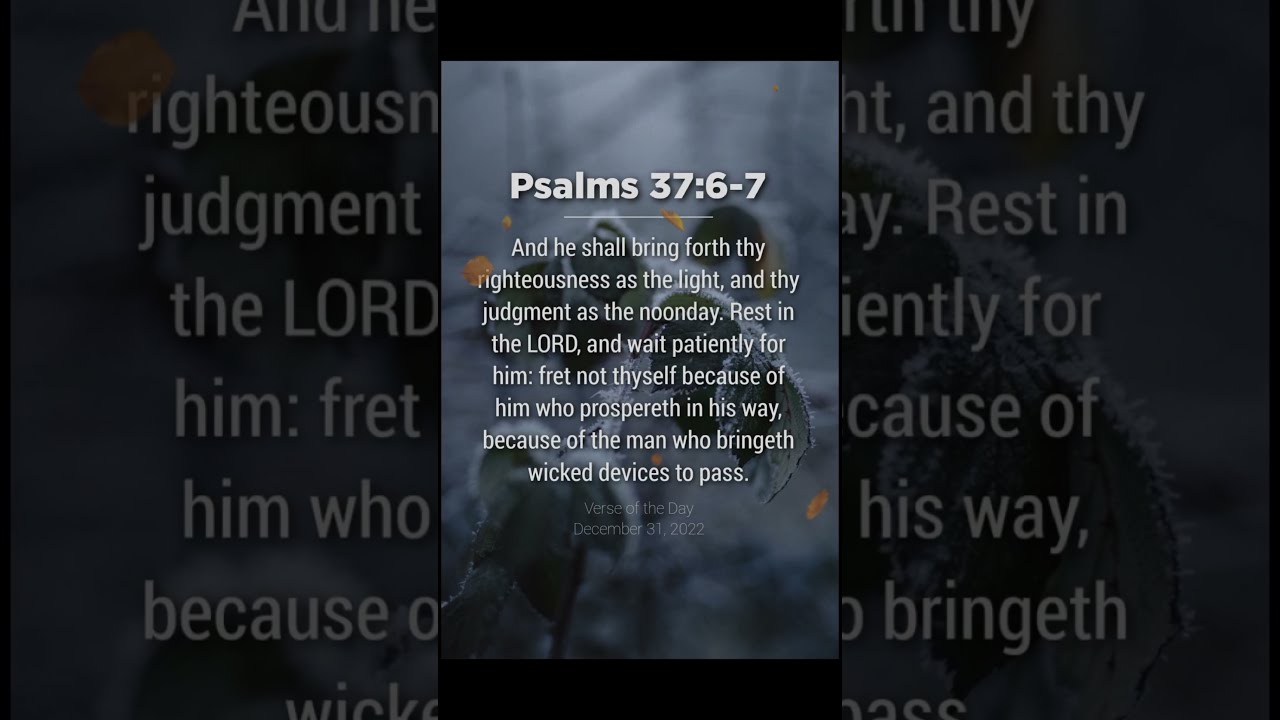This image features a Bible verse, Psalms 37:6-7, prominently displayed in bold white font. The verse reads: "And he shall bring forth thy righteousness as the light, and thy judgment as the noonday. Rest in the Lord, and wait patiently for him: fret not thyself because of him who prospereth in his way, because of the man who bringeth wicked devices to pass." The background is a grayscale, watermarked photograph of a plant, possibly covered in snow, giving a gloomy and serene atmosphere. The central portion of the image showcases the scripture text overlaid on the photograph, while the left and right sides display a zoomed-in and darkened version of the same plant image. Below the verse, in small, light font, it says "Verse of the Day, December 31st, 2022."